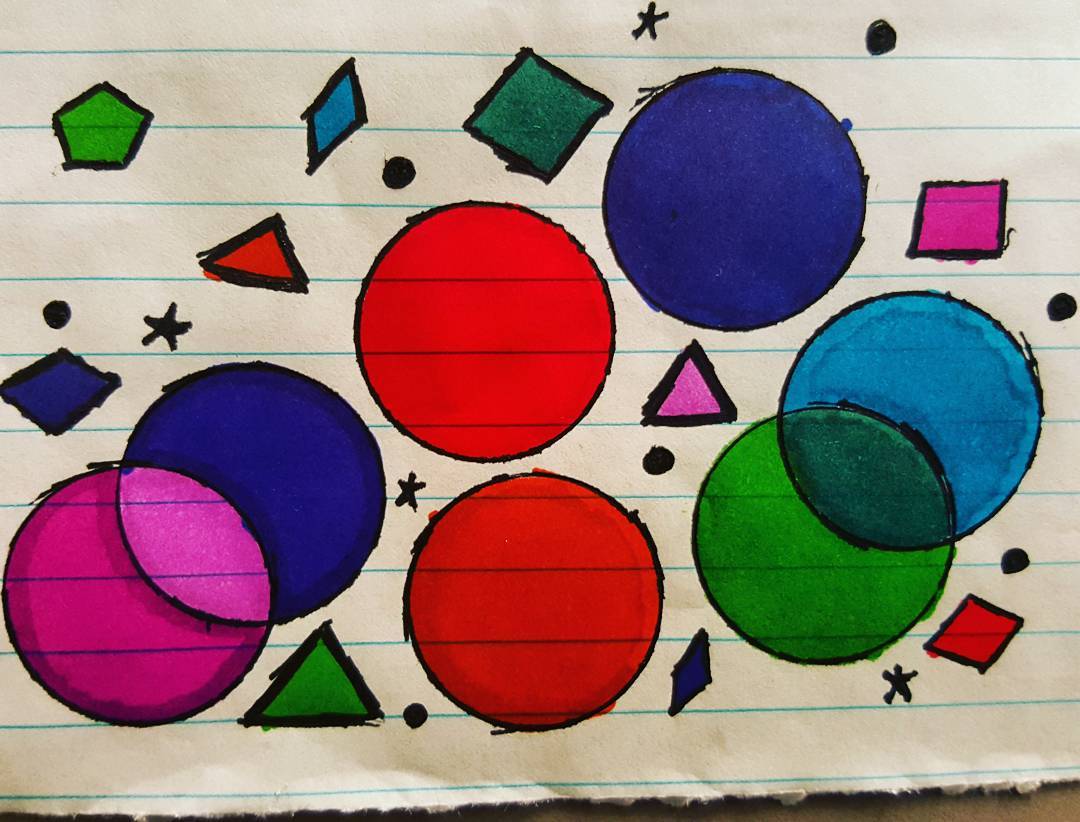This is a close-up photograph of a doodle on a slightly yellowed piece of notebook paper, characterized by parallel light blue horizontal lines and a torn bottom edge. The artwork features a variety of shapes, including circles, squares, triangles, rectangles, and diamonds, all drawn in vibrant colors such as red, blue, pink, green, purple, and brown. Among the most prominent shapes are seven large circles, with some intersecting pairs—such as the pink and blue circles forming a light pink intersection, and the blue and green circles creating a dark green overlap. The drawing also includes smaller geometric shapes like a green octagon, red and green triangles, a blue diamond, and several black star-shaped asterisks and dots scattered throughout. This colorful and detailed composition sits on a brownish surface, adding an additional layer of texture to the image.